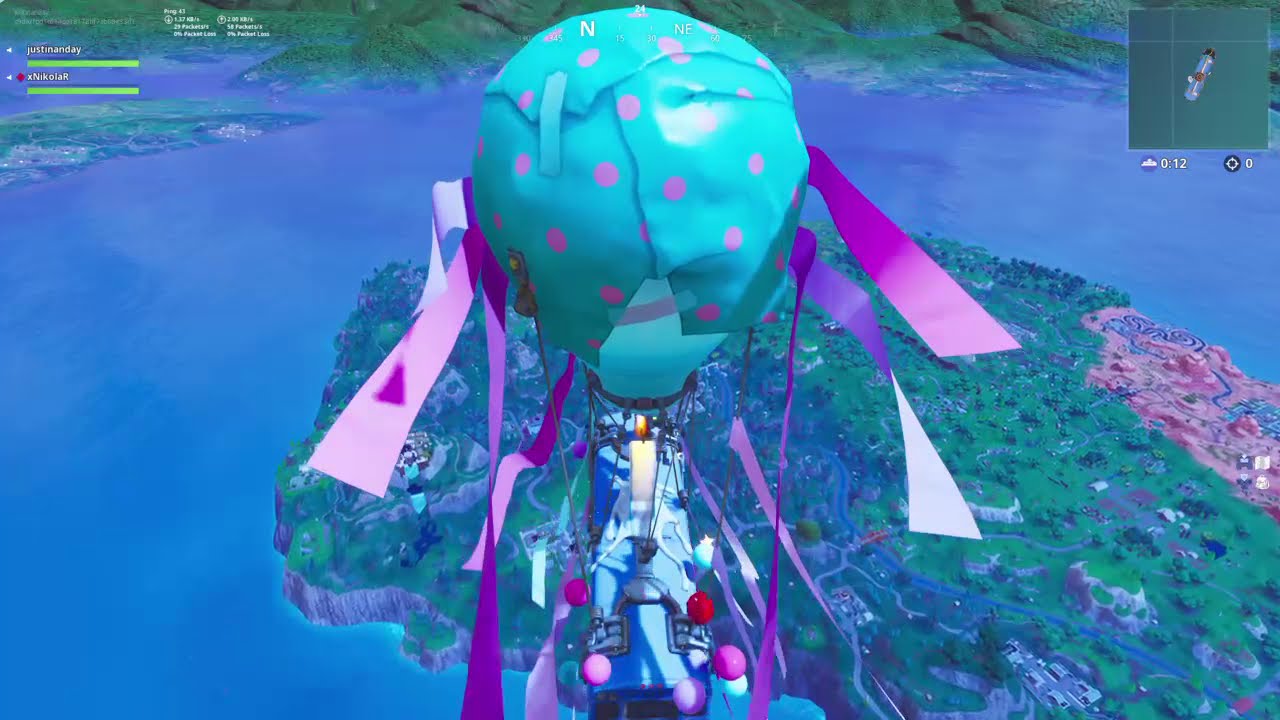The image is a clear, vibrant screenshot from the video game Fortnite, likely taken on a mobile device, console, or computer. Dominating the center is the iconic Fortnite battle bus, a blue vehicle suspended by a large light blue balloon adorned with pink polka dots, and trailing pink and purple ribbons. Hovering in the sky, it provides an aerial view of the expansive map below, which shows a large body of water with an island beneath, ready for players to dive into. In the top left corner, there are health bars and player names, specifically "Justin and A" and "xNicolar," along with some white text. The top right corner displays a radar-like mini map with a grid and a tiny depiction of the bus. The scene is richly colored with a palette that includes blue, green, red, light blue, pink, purple, gray, and black, all bathed in natural daylight, enhancing the vivid outdoor setting of the game environment.